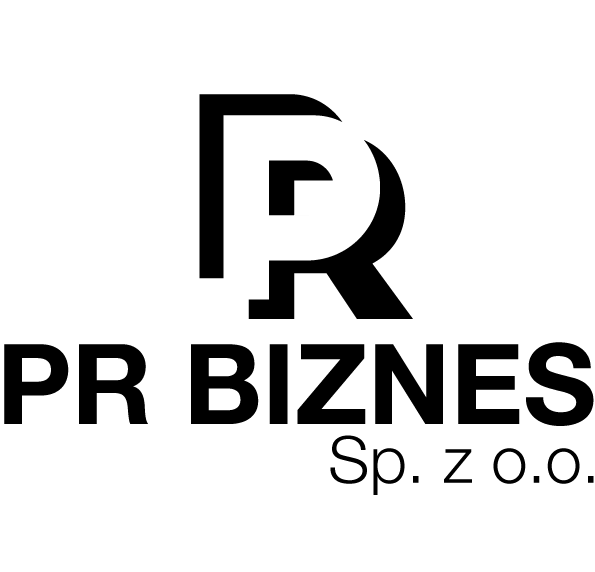The image features a clean, minimalist design set against a plain white background. Dominating the center is a large, stylized logo composed of a white 'P' overlapping a black 'R'. This creates a bold and visually striking 'PR' graphic. Directly beneath this logo, in uppercase black letters, are the words 'PR B-I-Z-N-E-S', clearly indicating the business name. Further below, in smaller, thinner black print, is the text 'S-p.Z.o.o.', where 'S' is capitalized and the rest are lowercase, each separated by a dot. The overall design is simple yet prominent, focusing solely on these textual and graphic elements.